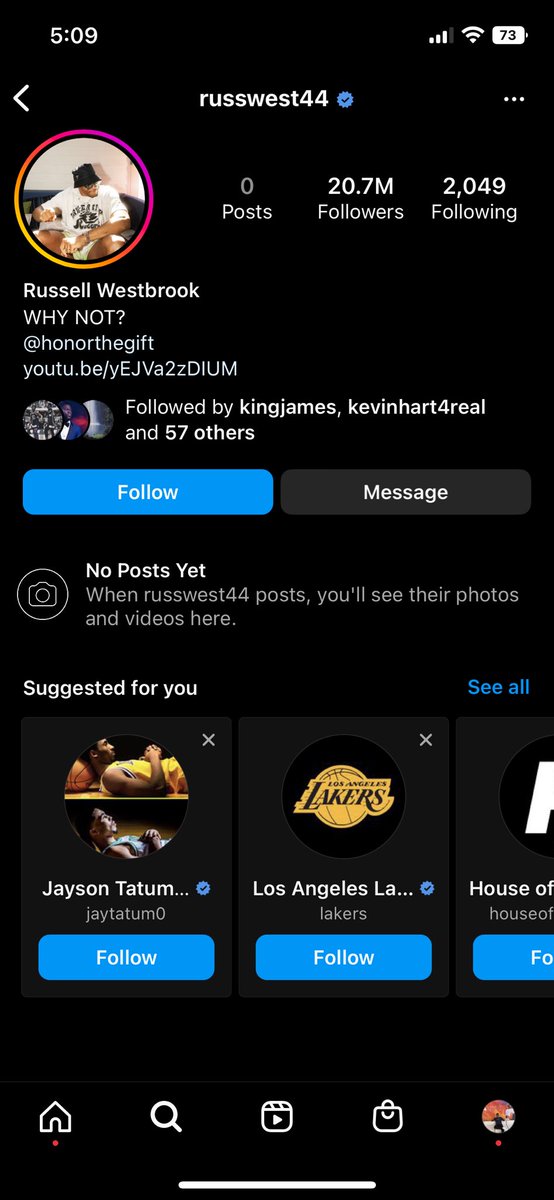The image depicts an Instagram profile page viewed on a smartphone. The account belongs to "rasswest44," which is verified, as indicated by the blue verification badge next to the username at the top. In the upper interface of the app, there's a back icon on the top left, along with the main Instagram icon on the top left and top right.

The profile has no posts, 20.7 million followers, and follows 2,049 accounts. On the left side of the screen, a profile picture displays a person dressed in white and wearing a black hat. The profile picture is encircled by a yellow and pink gradient, indicating an active story. Below the profile picture, the name "Russell Westbrook" is displayed, followed by the phrase "Why Not?" The bio contains a URL: "youtube.be/yejva2ztium". The profile is followed by notable individuals such as "Kim James," "Kevin Hart For Real," and 57 others.

Beneath the bio, there are two buttons: a blue "Follow" button on the left and a grey "Message" button on the right. Below these buttons, a message reads, "No posts yet. When rasswest44 posts, you will see their photos and videos here."

Further down, there's a section titled "Suggested for You" with a blue "See All" link and suggestions such as "Jason Tatum" (@jtatum0) and the "Los Angeles Lakers" (@lakers), represented by a yellow and black icon. Each suggestion includes a blue "Follow" button.

At the bottom navigation bar, there are icons for "Home," "Search," "IGTV," "Shop," and a "Profile" icon on the bottom right.